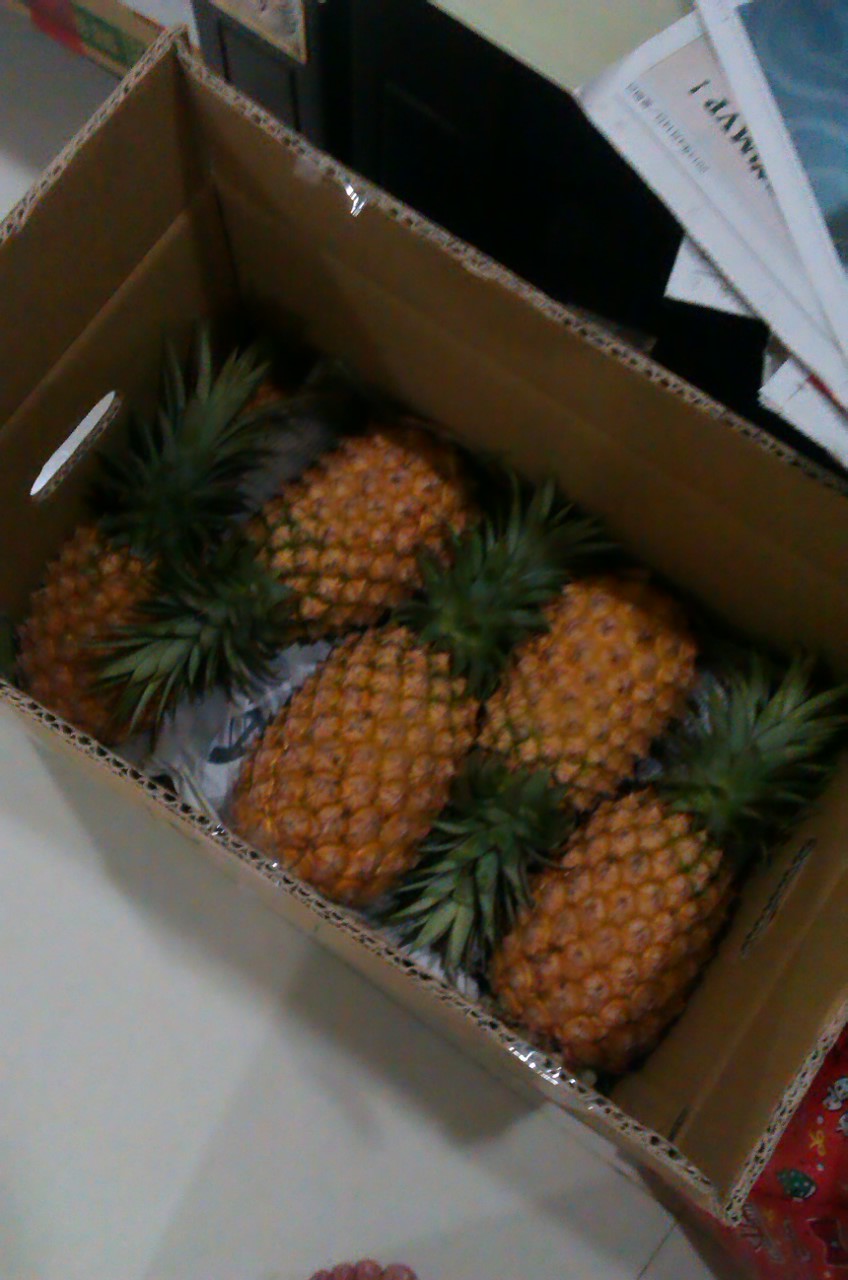This is a color photograph of a heavy-duty cardboard produce box filled with five whole pineapples. The box, which is positioned diagonally from the upper left to the lower right of the image, features carrying holes on either side for easy lifting. The box's four flaps are standing open, revealing remnants of clear tape along the edges. Inside, the pineapples alternate in orientation: one faces down, the next up, and so on, with their orange-gold bodies and green crowns clearly visible.

At the upper right of the photo, just outside the box, there is a newspaper written in a foreign language, slightly fanned out. The box rests on a white surface, with some red festive-print paper in the lower right corner. There are also visible toes at the very bottom center of the frame, suggesting the presence of a person nearby.